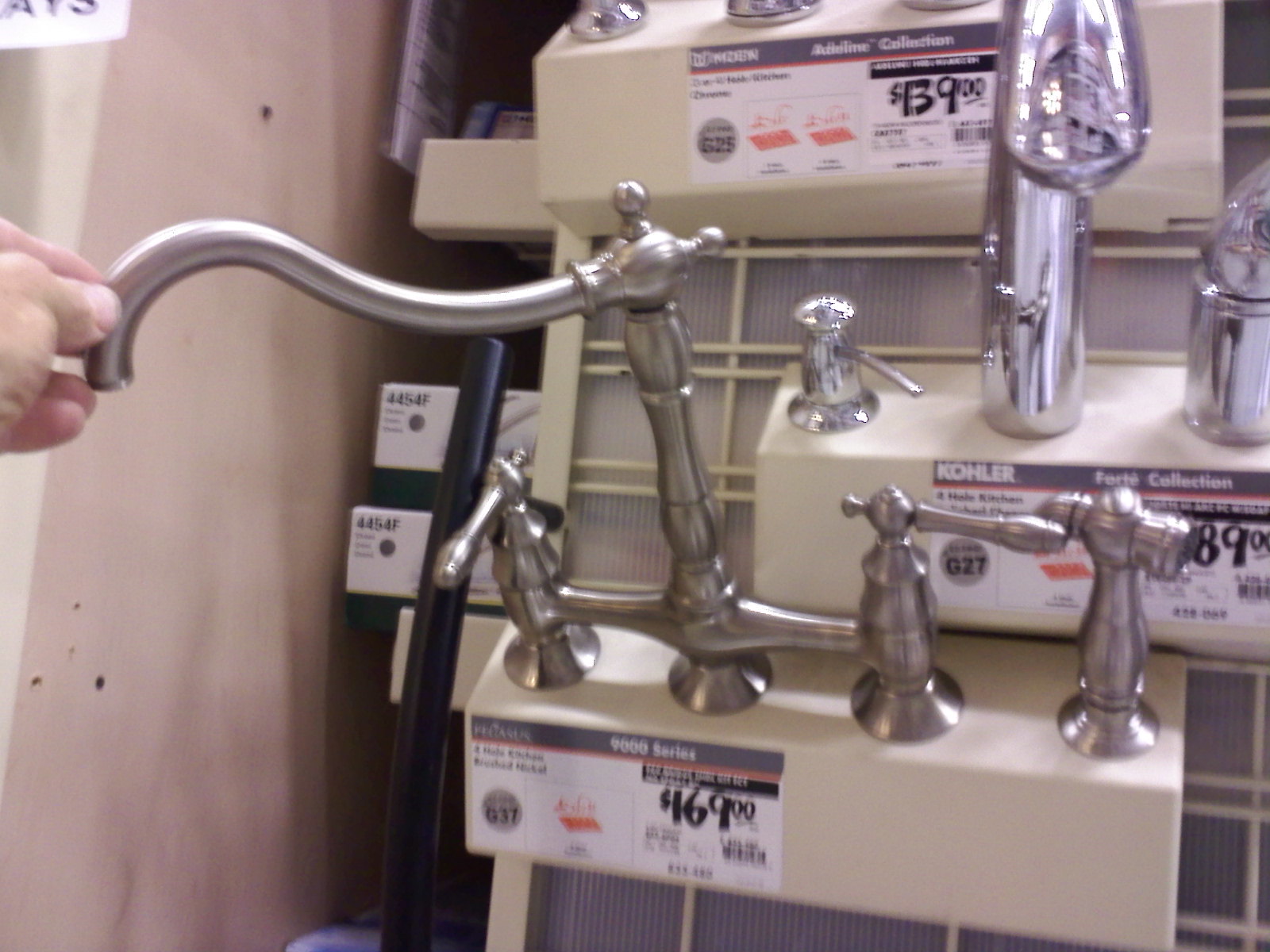This detailed photograph captures a display of high-arch kitchen-style faucets inside what appears to be a Home Depot store. The faucets, predominantly featuring a nickel or stainless steel finish, include brands such as Kohler and Mohn. The display is set against a wooden backdrop with visible price labels, although some are partially covered. The most prominent faucet in the image is priced at $169 and bears the Kohler name. This faucet is being touched by a white male hand, which is turning the spout, seemingly testing its action. Additionally, there are other faucets displayed with price tags of $139 and $189. The faucets boast dual handles and a veggie sprayer option, underscoring their kitchen utility.